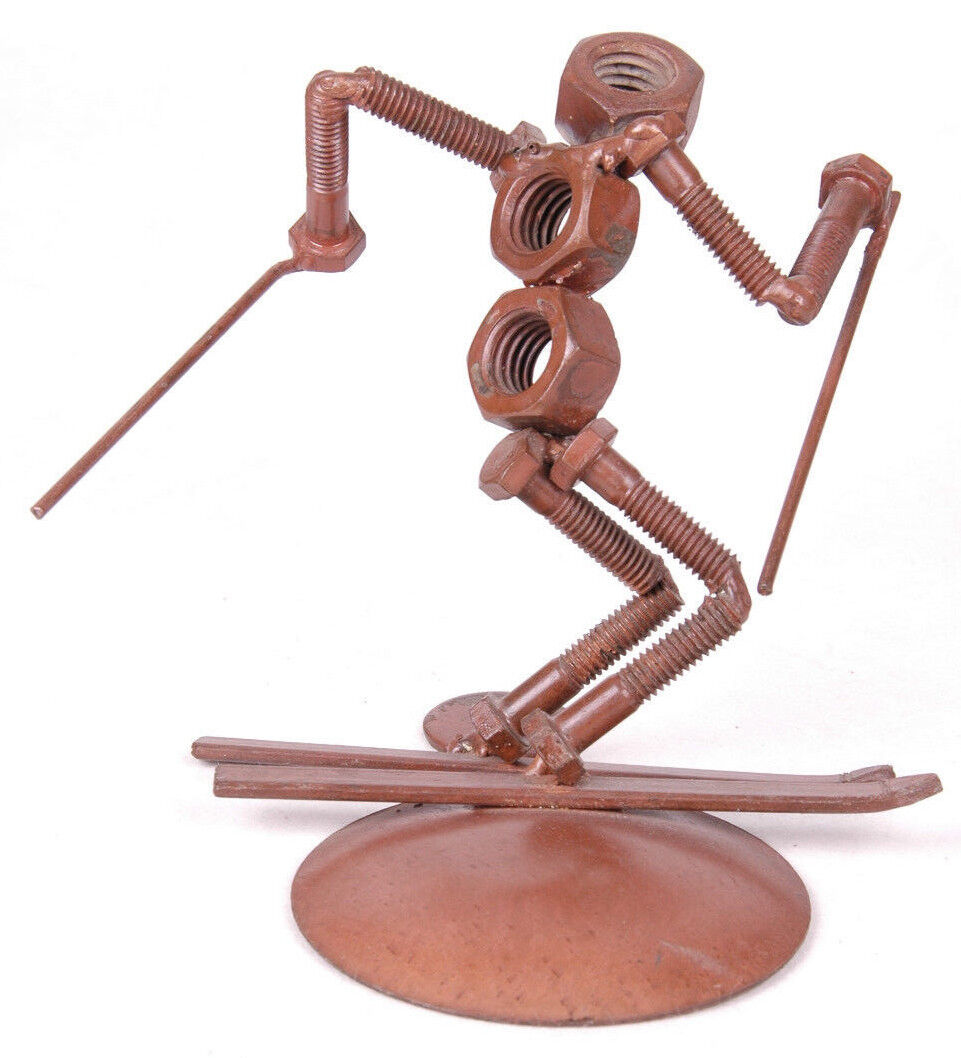The image depicts a detailed miniature sculpture made from various nuts, bolts, and screws, cleverly welded to resemble a man skiing. The sculpture is painted in a bronze color and is mounted on a small, circular bronze-colored base. The skier's head is fashioned from a single bolt, while two bolts are used to create the torso. The arms and legs are made from bent screws, with the arms appearing to hold ski poles formed from elongated nails. The knees are articulated with precise welding, giving the illusion of a skier in motion. The skis themselves are crafted from two long, flat metal pieces, securely attached to the screws that form the legs. This intricate assembly of everyday hardware presents a dynamic and lifelike representation of a skier in action.